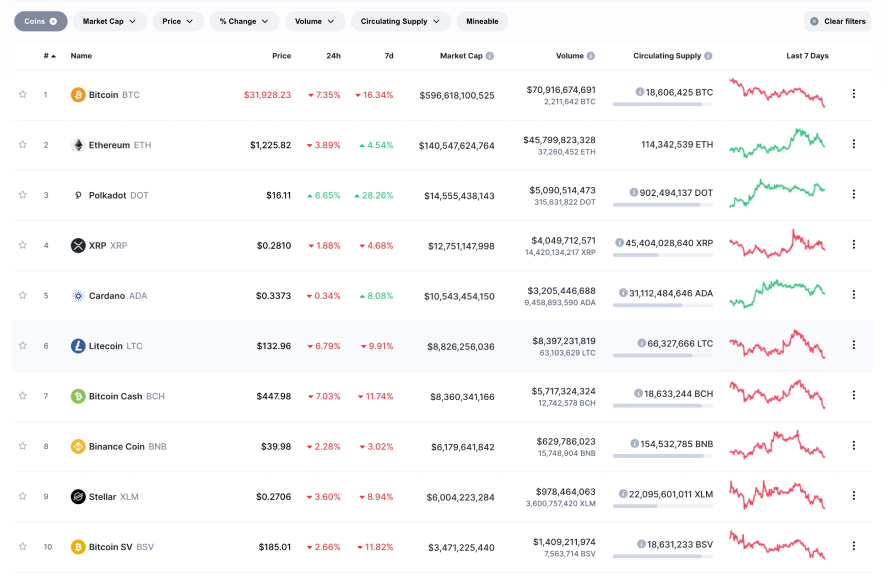In the image, we see a screenshot displaying financial information focused on cryptocurrency. The interface is well-structured, beginning at the upper left corner with various interactive buttons labeled "Coins," "Market Cap," "Price," "Change," "Volume," and "Circulating Supply," each accompanied by a drop-down menu. Positioned to the right of these buttons is the label "Mineable."

Below these tabs, a series of columns are presented with clear headings aligned from left to right. These headings are "Name," "Price," "24h," "7d," "Market Cap," "Volume," "Circulating Supply," and "Last 7 Days." The first entry in these columns is "Bitcoin," identified by its distinctive 'B' icon.

Bitcoin's financial details are listed across the adjacent columns. The current price is shown as $1,928.23, marked by a red downward arrow indicating a 7.35% decrease over the past 24 hours and a more severe 16.34% drop over the past seven days. Accompanying these figures is a small red chart under the "Last 7 Days" column, graphically representing Bitcoin's downward trend during the week, highlighting the cryptocurrency's declining cycle over recent days.